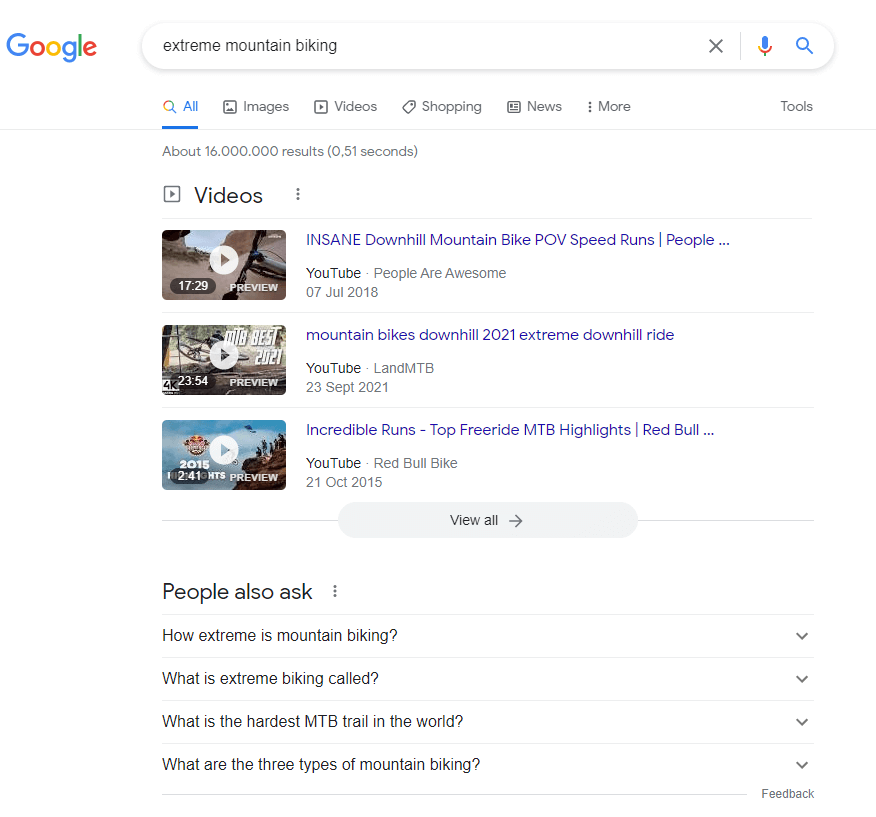A screenshot of a Google search result page is displayed, featuring the well-known colorful Google logo at the top. The search query entered is "Extreme Mountain Biking," visible within the search box. To the right of the search box, there are icons for a colorful blue and red microphone and a blue magnifying glass. Below the search bar, various navigational tabs are present, including "All," "Images," "Videos," "Shopping," "News," and "More." The "All" tab is highlighted with a blue underline, indicating it is currently selected. Adjacent to these tabs is a "Tools" button.

The search results begin with a dedicated video section showcasing three YouTube video thumbnails and their titles, all in clickable blue text for user interaction. The first video is titled "Insane Downhill Mountain Bike POV Speedruns," the second is "Mountain Bikes Downhill 2021 Extreme Downhill Ride," and the third is "Incredible Runs Top Freeride MTB Highlights Red Bull."

Following the video section, there is a "People Also Ask" feature containing commonly queried questions related to extreme mountain biking. The questions listed include "How extreme is mountain biking?", "What is extreme mountain biking called?", "What is the hardest MTB trail in the world?", and "What are the three types of mountain biking?" Each question is accompanied by a small downward arrow, allowing users to expand and view detailed answers.